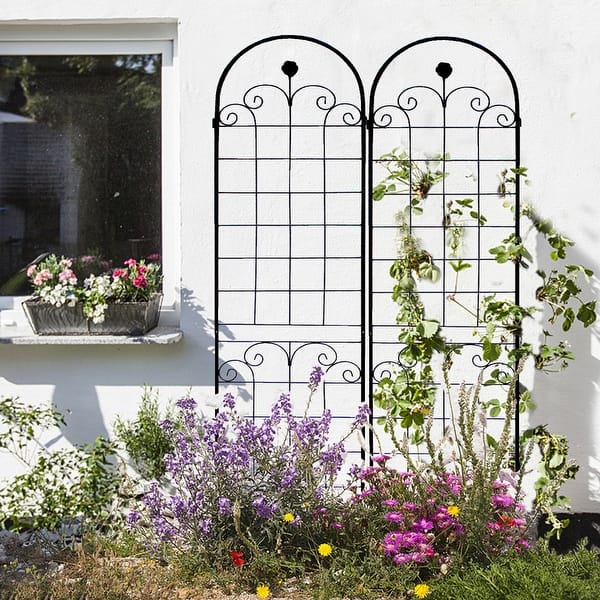The photograph captures a quaint and colorful flower garden nestled against a white stucco house. Centered in the scene are two elegant black wrought iron trellises with arched tops and decorative curled elements, one of which supports a vibrant green vine climbing nearly to the top. At the base of these trellises, a burst of bright flowers—pink, yellow, purple, and some dandelions—adds a lively palette to the garden. To the left of the trellises is a window with a ledge, adorned with a planter box full of impatiens in shades of white, light pink, and dark pink. Despite an unkempt appearance, the garden exudes natural beauty, accentuated by the warm, sunny day casting bright shadows across the scene.